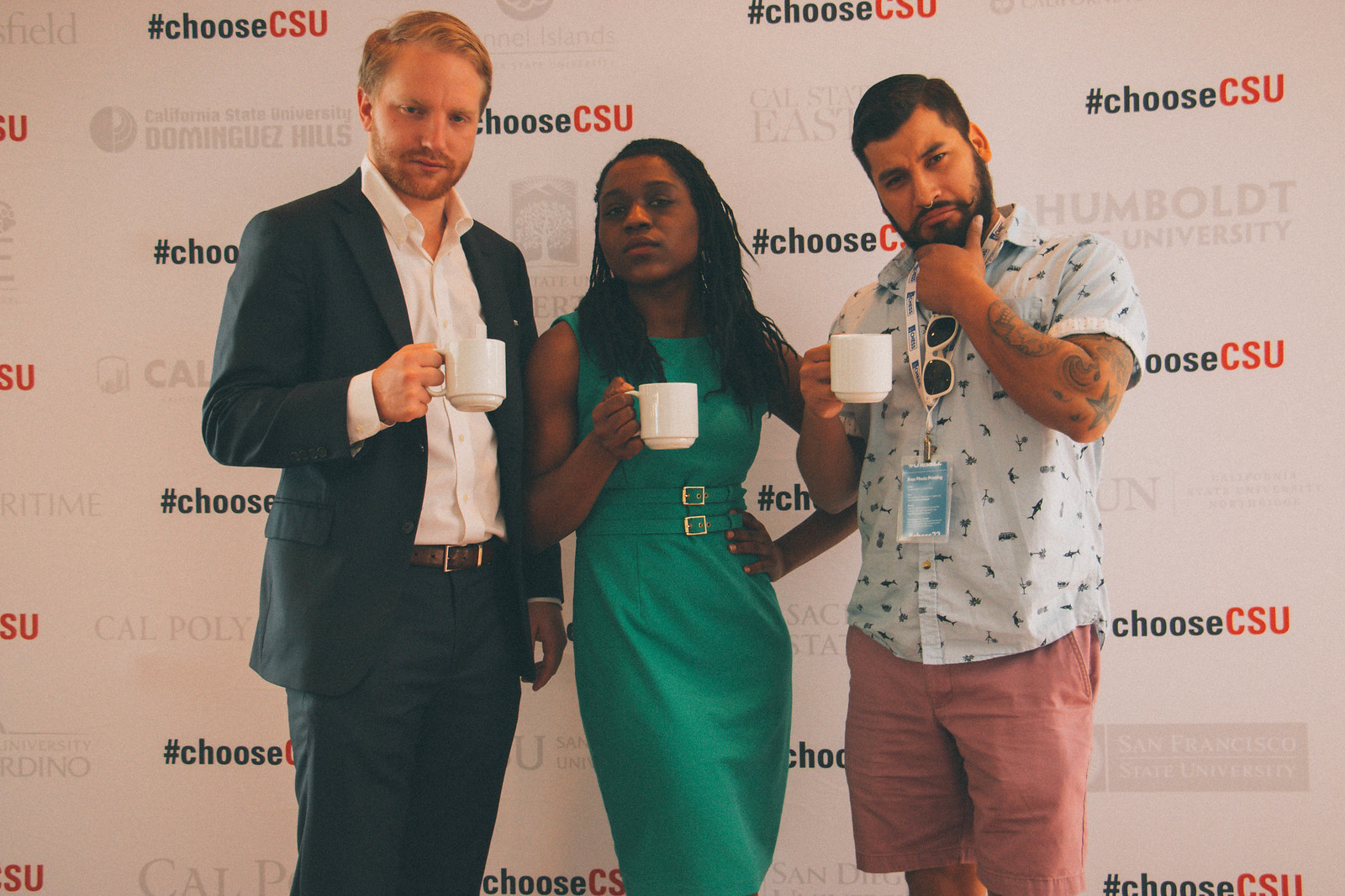The image features three individuals standing in front of a step-and-repeat backdrop adorned with numerous university logos and slogans such as "#chooseCSU," "California State University," "Dominguez Hills," "Cal Poly," "Humboldt University," "Cal State East," and "San Francisco State University." The repeated logos are predominantly in gray and black, with "CSU" highlighted in red.

From left to right, the first person is a young man with reddish-blonde hair and a short beard, dressed in a dark suit with a white button-up shirt but no tie. He holds a white coffee cup in his hand. 

In the middle, a shorter African American woman with long, dark braids sports a sleeveless, belted green dress. She, too, holds a white coffee cup and looks directly at the viewer.

On the right, another gentleman with dark hair, a beard, and a mustache is dressed in a casual, printed short-sleeve button-up shirt and peach-colored shorts. He has a lanyard with an ID badge and white sunglasses hanging around his neck, along with tattoos visible on his left arm. He also carries a white coffee cup.

All three strike a posed and somewhat pensive expression as they face the camera.